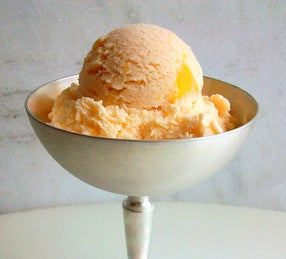The image is a small, square-shaped picture without a border, featuring an elegant, elevated dessert bowl that has a frosted grayish exterior with a darker, silver-colored rim and a metallic, copper-colored, and reflective interior. The stem of this bowl is partially visible, suggesting it sits on a white, rounded surface. The bowl contains a large, round scoop of creamy vanilla ice cream with an orangish hue, likely indicating a blend of peach or sherbet. A noticeable chunk of what appears to be an orange or peach is embedded in the ice cream on the right side of the scoop. The background presents a marbled gray and darker gray wall that appears slightly blurred, hinting the photo might have been taken indoors, possibly for a food display on a website like Grubhub or Uber Eats.